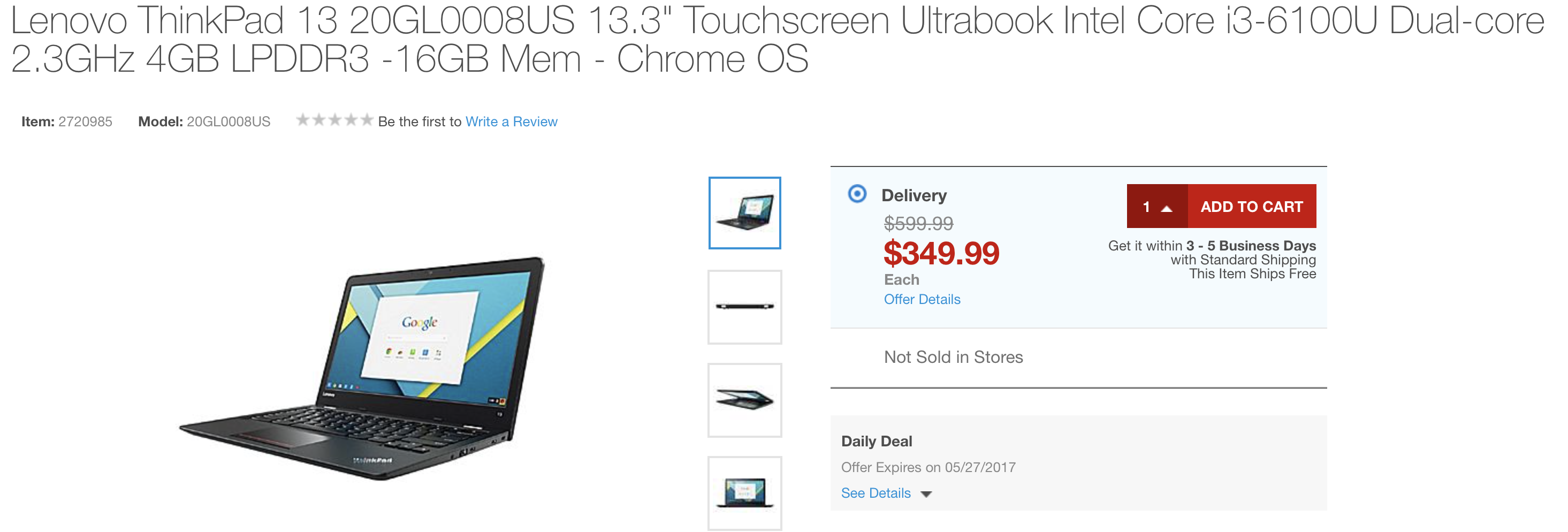This is a detailed screenshot from an electronic shipping website, specifically featuring a product page for a Lenovo ThinkPad 13 Chromebook (Model: 20GL0008US). The image shows a close-up view of the page without revealing the browser or computer type used to capture it. At the top, the product title is displayed in light grey text: "Lenovo ThinkPad 13, 20GL0008US, 13.3 inches touch screen ultrabook, Intel Core i3-1610U dual-core 2.3GHz, 4GB LPDDR3, 16GB memory, Chrome OS." 

Below the title, smaller text lists the item number, model number, and a five-star rating indicator. Beneath this information is a photo of the Chromebook itself, which is a black laptop with a blue pattern, shown open with its desktop visible. The desktop displays a browser window with Google open against a blue background with a yellow pattern.

To the right side of the laptop image, purchase details are provided. A blue rectangle with black text reads “Delivery.” The original price of $599.99 is crossed out and replaced with a sale price of $349.99 in red lettering. Next to the price is a red rectangle indicating "Add to Cart" with a number one inside it. Below this, the text confirms, “Not sold in stores.”

To the left of the price information, there are four smaller images of the laptop, showing various angles: fully open, slightly open, and open towards the viewer.